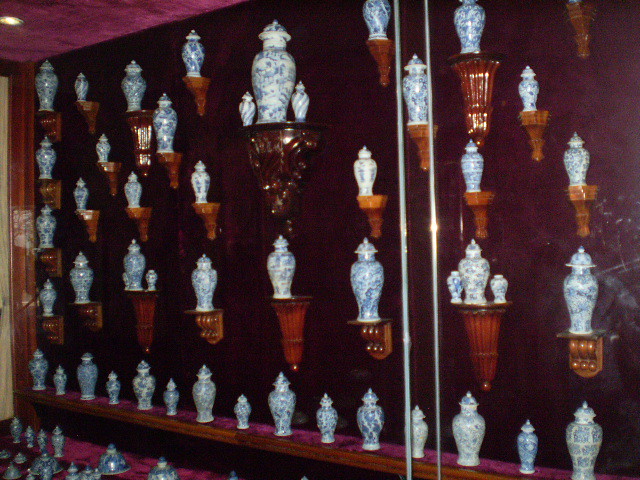The image depicts an indoor scene with subdued lighting, showcasing a large glass case featuring a series of brown wooden shelves, some built into the case itself and some resembling sconces. Each shelf delicately holds a collection of vases that vary significantly in size, from very tiny to quite large, making them appear like urns. All the vases share a consistent color scheme of blue and white, with intricate, swirling patterns. The case is designed with a brown framework and includes small holders that securely rest each vase. The upper left corner of the image captures a striking detail: a velvet-textured red-purple element which matches the color at the top edge of a shelf inside the glass case, extending to a similar hue outside the case. Additionally, in the bottom-left corner, there’s a row of vases arranged in an alternating pattern of large and small sizes. This careful arrangement enhances the display of these exquisite, blue and white porcelain pieces, creating an elegant visual symphony.